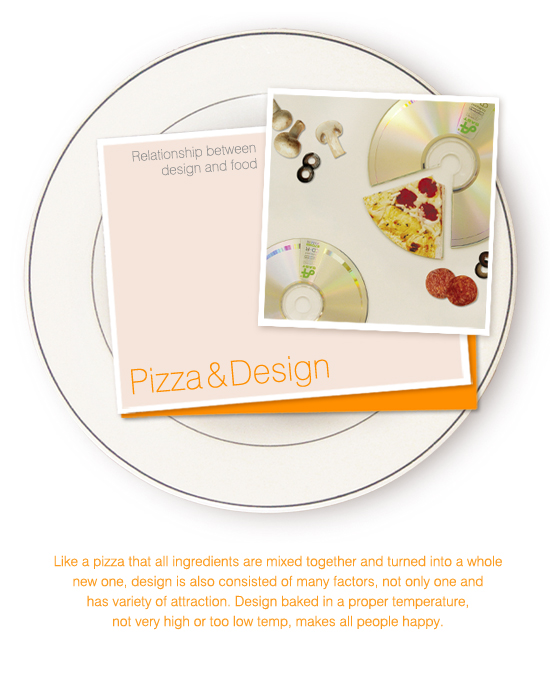The image is a detailed digital flyer set against a clean, white background. At the center of the flyer is a top-down view illustration of a white dinner plate that has a thin black line outlining its outer rim and a thinner gray line forming a concentric circle closer to the center. Laying on the plate are two overlapping pieces of paper; the bottom one, which is only partially visible, is a dark orange color, while the top one is a pale orange color with a white border. 

On top of these papers is a square piece of paper featuring a striking image of a CD with a pizza slice cut out of it, revealing pepperoni, olives, and mushrooms. In the upper left of this square, there is the black letter '8' accompanied by whole white mushrooms tinged with brown. The top piece of paper reads "relationship between design and food" in light blue-gray lettering, with larger gold letters at the bottom stating "pizza & design."

Beneath the plate, there is an informative paragraph in orange font. It reads: "Like a pizza that all ingredients are mixed together and turned into a whole new one, design also consists of many factors, not only one, and has a variety of attractions. Design baked at a proper temperature, not too high or too low, makes all people happy."